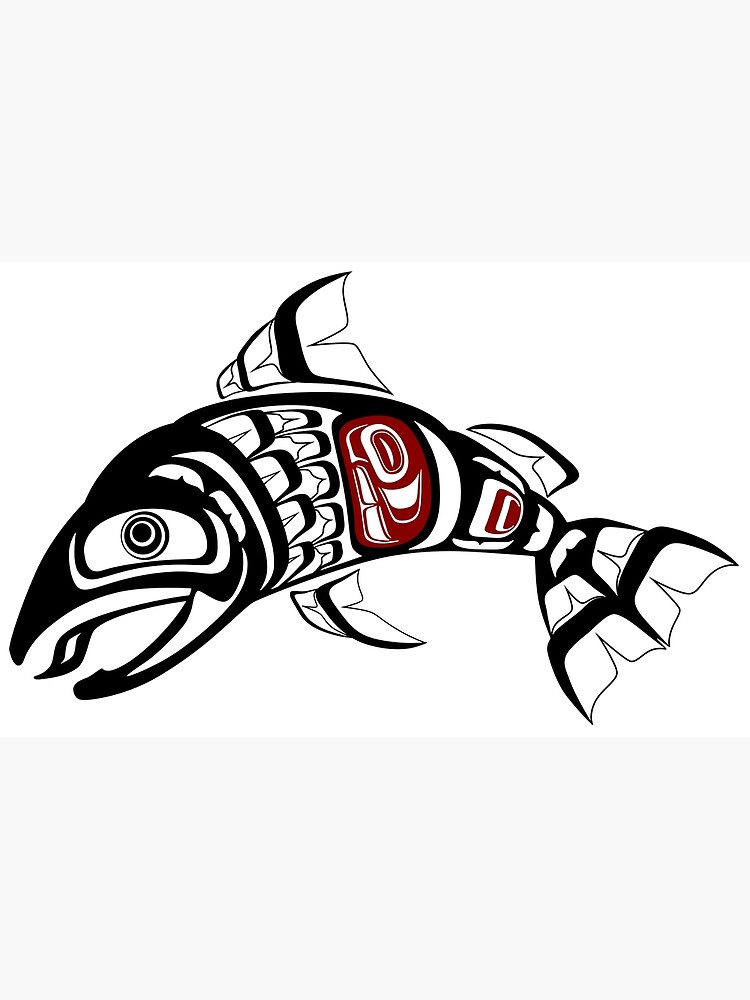This is a very detailed, abstract drawing of a fish rendered in black and white, with eye-catching accents in crimson red. The fish faces to the left and is depicted in a mixture of loose, broken-up shapes, giving it a hand-drawn, almost caricature-like appearance. The composition features the fish curving gracefully, almost in a semi-circle, with sharp fins extending from its body. These fins showcase bold black stripes. Surrounding the image is a large rectangle with a white border set against a gray background.

The fish's body is predominantly black with white scales outlined in black. Notable details include lines around the eye and distinct gills, all drawn with either black or white space. A significant crimson red oval area is positioned just behind the gills, followed by another similarly colored rectangular rounded shape, adding a splash of color to the monochromatic theme. The design hints at a Japanese stylistic influence and an artistic, tribal-like line art approach. The fish appears to be smiling, accentuating its whimsical nature.